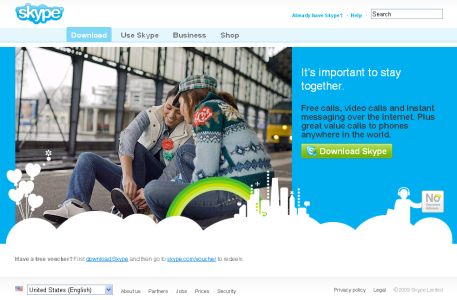The image features a promotional advertisement for Skype prominently displayed at the top of the page. The classic Skype logo, a cloud with an 'S' in the middle, is clearly visible. Below the logo, text encourages users to "Download, Use Skype for Business, Shop". In bold, compelling letters, the ad emphasizes, "It's important to stay connected," highlighting the service's offerings of free calls, video calls, and instant messaging over the internet. Furthermore, it promotes great value calls to phones anywhere in the world.

A green button labeled "Download Skype" is featured, inviting users to take action immediately. 

In the primary image, two women, who appear to be friends, are sitting together at a train station with a train visible in the background. Their relaxed posture suggests they are comfortably waiting, possibly using Skype to pass the time or stay connected with loved ones. The overall scene portrays a seamless blend of human connection and technological convenience.